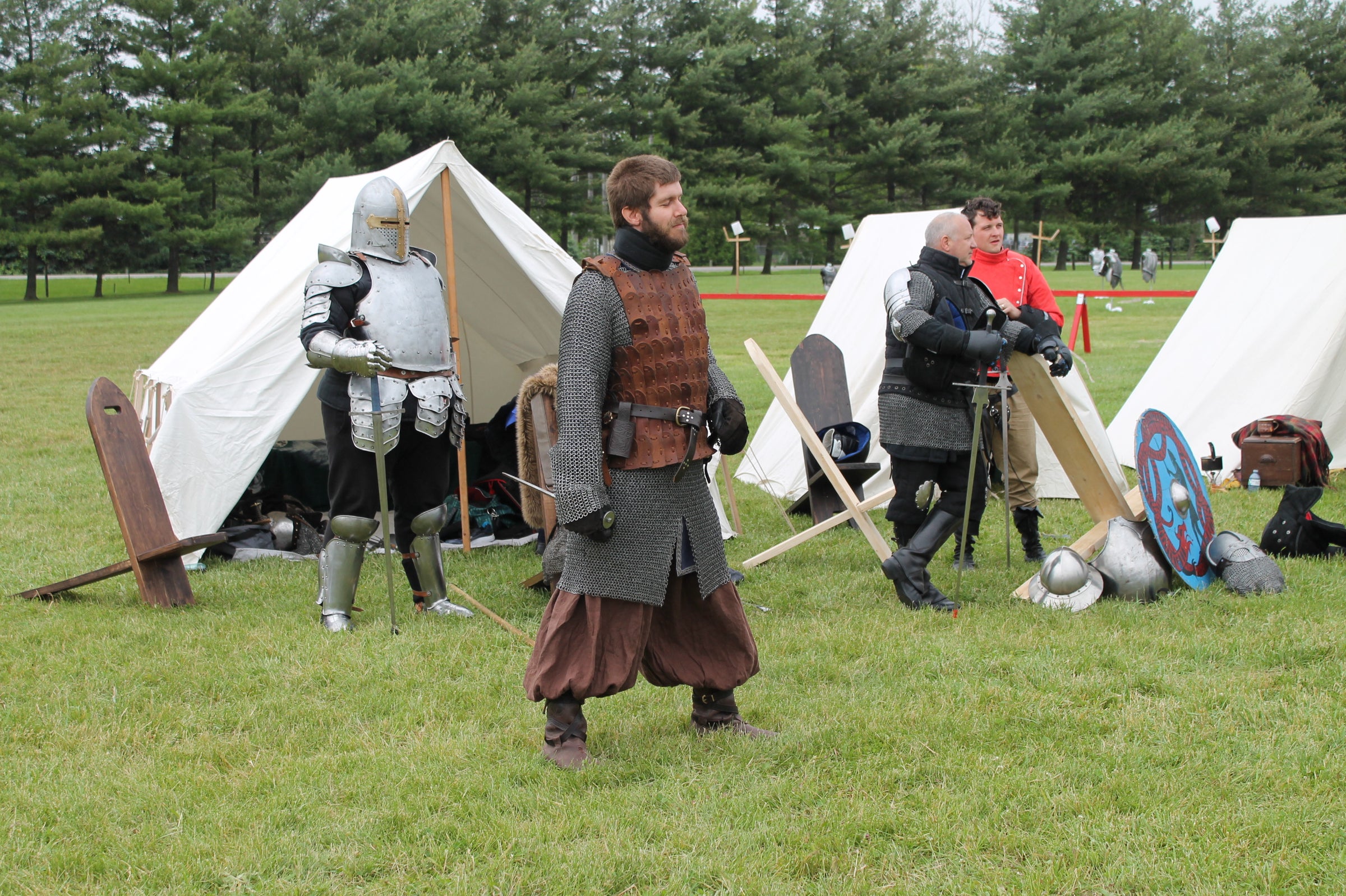This is a color photograph in landscape orientation, depicting several costumed actors at a Renaissance festival or fair situated in a large grassy field under a sunny daytime sky. The foreground features four men standing in front of three white canvas tents, reminiscent of medieval shelters with simple wooden frames. 

**From Left to Right**:
- The man on the far left is clad in full silver body armor, including a helmet that conceals his face, and he holds a sword.
- Next to him is the central figure, a young man around 30 years old, in a detailed costume comprising a brown leather vest, gray chain mail shirt, puffy brown pants, and brown boots. He has light brown short hair, a beard, and wears black gloves, a waist belt, and a high-neck garment designed to protect his throat. He appears to be holding a spear or dagger.
- On the right side, two additional men are dressed—one in body armor similar to the knight, and another in an orange tunic paired with brown pants. These two are gazing into the distance in front of what looks like an archery target.

Scattered around the characters are various pieces of medieval-themed accessories, including shields and other armor components. 

In the background, a red makeshift fence, fashioned from a ribbon, cordons off an area. Beyond this, a line of dense, dark green pine trees forms the backdrop. Across a street behind this line of trees, the sky is visible, adding depth and a sense of realism to the photograph. Further into the distance, additional figures in period attire can be seen, though their details are indiscernible.